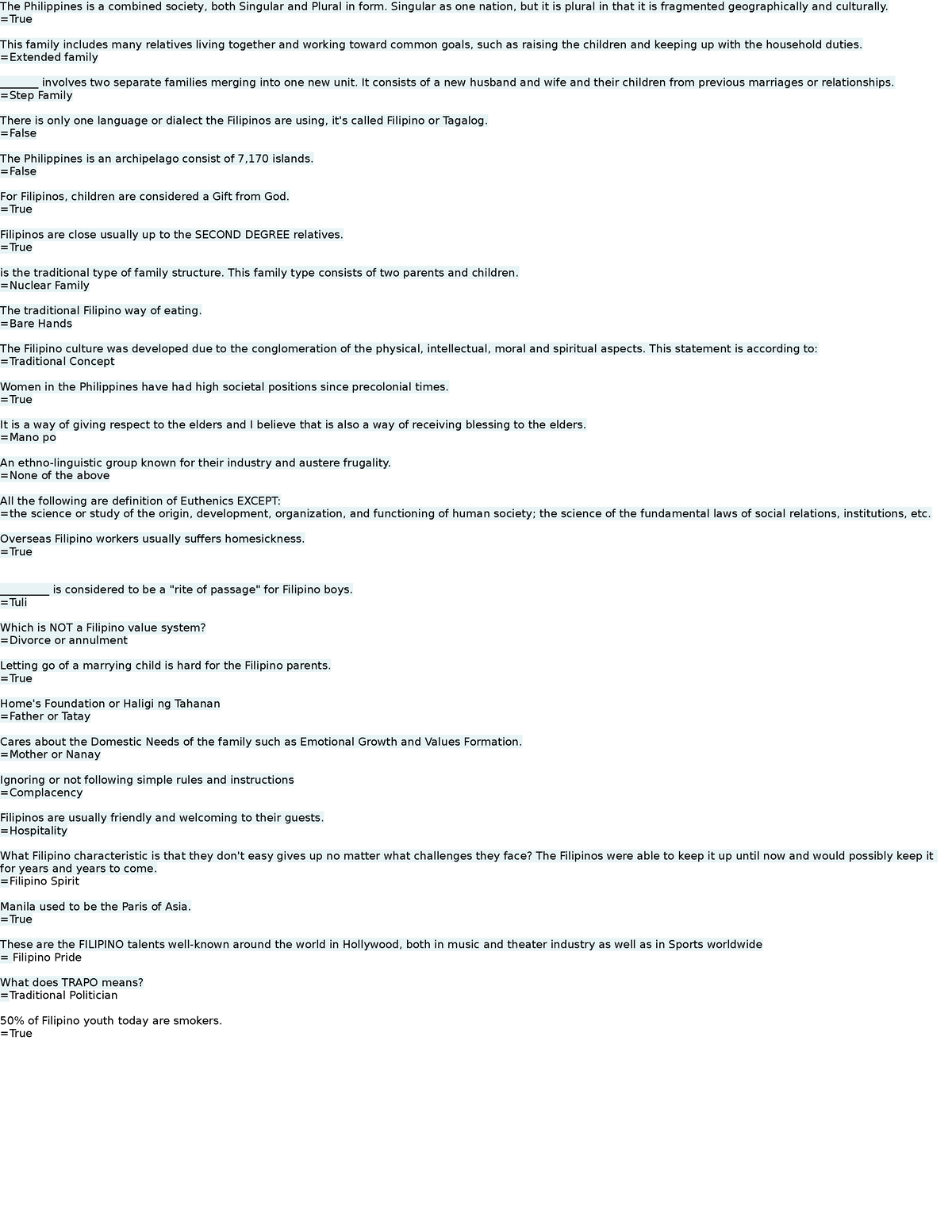**Website Information on Filipino Society and Family Structures**

The Philippines is a unique society that is both singular and plural in form. Singular as one nation, it is plural due to its geographical and cultural fragmentation. Filipino families often include numerous relatives living together and collaborating to achieve common goals, such as raising children and maintaining household responsibilities; this is indicative of an extended family system.

The information provided appears in a question-and-answer format. It covers different types of family structures:

1. **Extended Family**: This family type includes many relatives who live together and work towards common goals, like child-rearing and household upkeep.
2. **Step Family**: This involves two separate families merging into one new unit, consisting of a new husband and wife and their children from previous marriages or relationships.
3. **Nuclear Family**: The traditional family structure in the Philippines, which consists of two parents and their children.

Additionally, the information corrects some misconceptions:
- There is not only one language or dialect spoken in the Philippines; the primary languages are Filipino and Tagalog, but many other dialects are spoken across the archipelago.
- The Philippines is composed of approximately 7,641 islands, not 7.17.
- Filipinos traditionally view children as a gift from God, emphasizing the cultural and familial importance of offspring.

The traditional Filipino way of eating often involves using bare hands, which is a cultural practice still observed in many households.